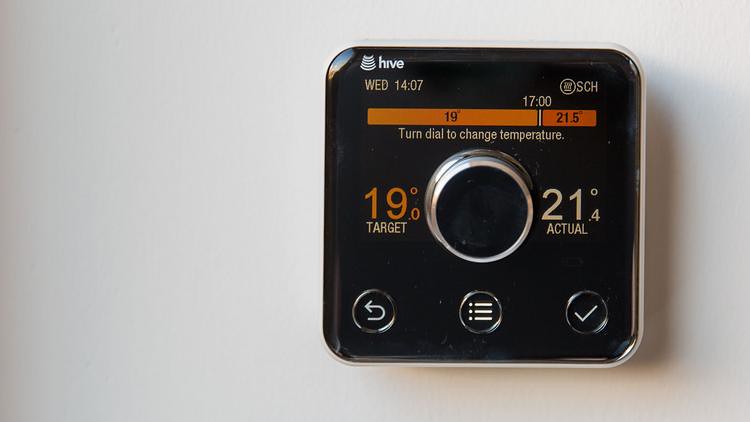This color photograph showcases a black, square-shaped control panel set on a grayish-white surface. Central to the panel is a silver-surrounded round knob, which functions as a dial. Above the dial, instructions are inscribed in white text against the black background: "Turn dial to change temperature." Immediately above this text, an orange horizontal bar transitions from a lighter shade on the left to a deeper, richer orange on the right. To the left of the dial, the target temperature is displayed as "19 degrees," while "21.4 degrees actual" is indicated to the right, reflecting the current temperature. The numbers "19" and "21.5 degrees" are also displayed on the respective sides of the orange bar, correlating with the gradient. In the upper left corner of the panel, the word "Hive" is prominently displayed, likely representing the brand name, along with its associated logo. The control panel casts a faint shadow to the right, adding a subtle depth against the gray surface.